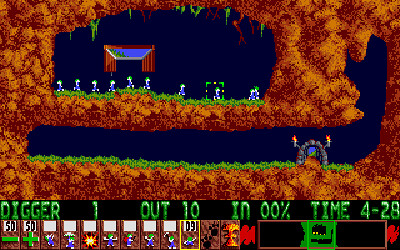In this screenshot from a video game, the scene is set underground within a maze-like cave. The environment is characterized by reddish-brown dirt layers with patches of green grass and flowers. The upper level features a blend of dirt and vegetation, while below it, there's an arched stone doorway partially enveloped by the ceiling. Moss, branches, and roots dangle from above, adding to the cavernous atmosphere. The background is dark, with a window-like structure framed by brown curtains.

Nine characters, each dressed in blue overalls and sporting green hair, are navigating the maze. Aiming to accomplish specific missions, these characters are displayed along the bottom of the screen, labeled as "Duder 1/10: 0.00% Time - 4:28." Additional icons illustrating different actions or items, such as a horizontal green bar, a green cross, an umbrella, an explosion, outstretched hands, a scarf, a fist, a pickaxe, and others, are also visible. Finally, a map section is highlighted by a green square, indicating the current location within the game.